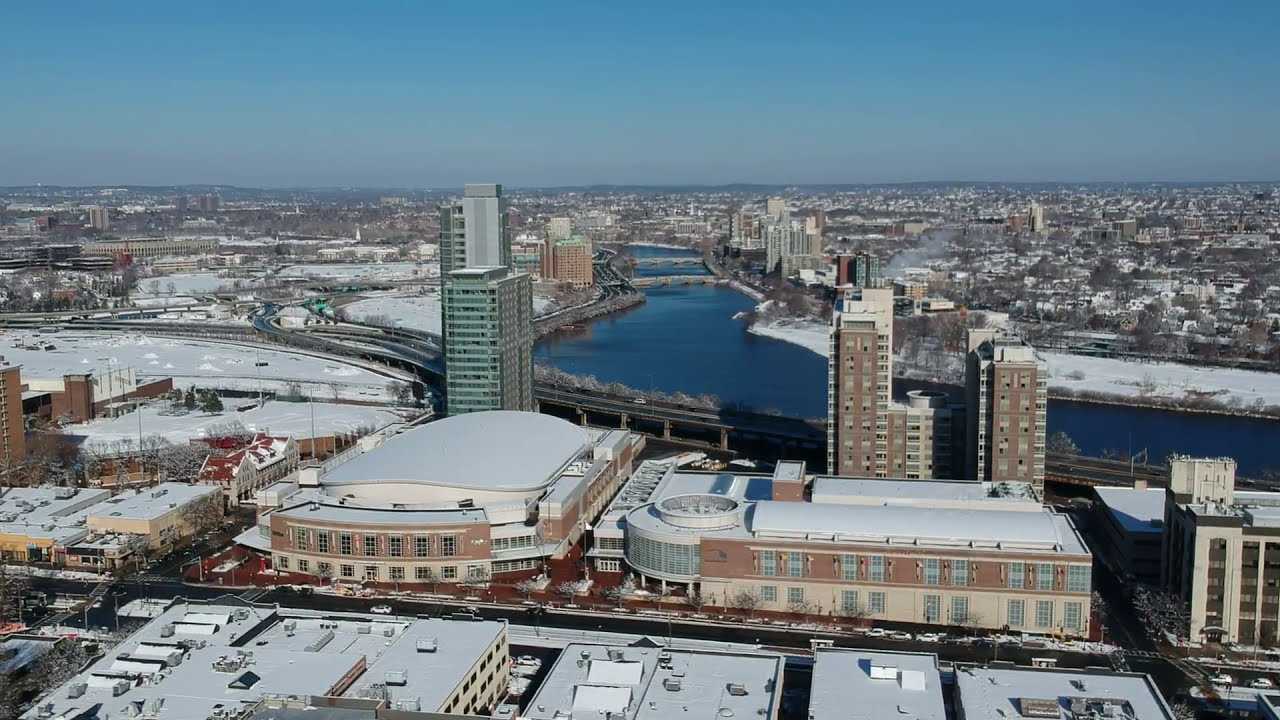The image displays an aerial view of a city in the wintertime, showcasing a snow-covered urban landscape. In the foreground, there are large, broad buildings resembling stadiums or arenas, their rooftops blanketed in white. Moving further back, you notice the cityscape populated with gray, flat rooftop structures, intermittently dotted with white patches of snow. Notably, two side-by-side brick buildings, with distinctive red and white facades, stand out prominently. A river, vividly blue and partially frozen, bisects the city, winding sinuously from the right side of the image towards the center, then curving off to the left. This waterway is spanned by small bridges and flanked by tall buildings along the riverfront. Beyond the river, the view extends to a sprawling collection of smaller structures, indicating a large cityscape. In the distance, skyscrapers rise, suggesting a bustling metropolis with more buildings receding into the horizon. The scene is set against a gradient sky, transitioning from light blue at the bottom to a deeper blue at the top, enhancing the chilly, serene ambiance of the winter day. Leafless gray trees add to the stark, wintry feel of the image, emphasizing the pervasive blanket of snow that covers the entire city.